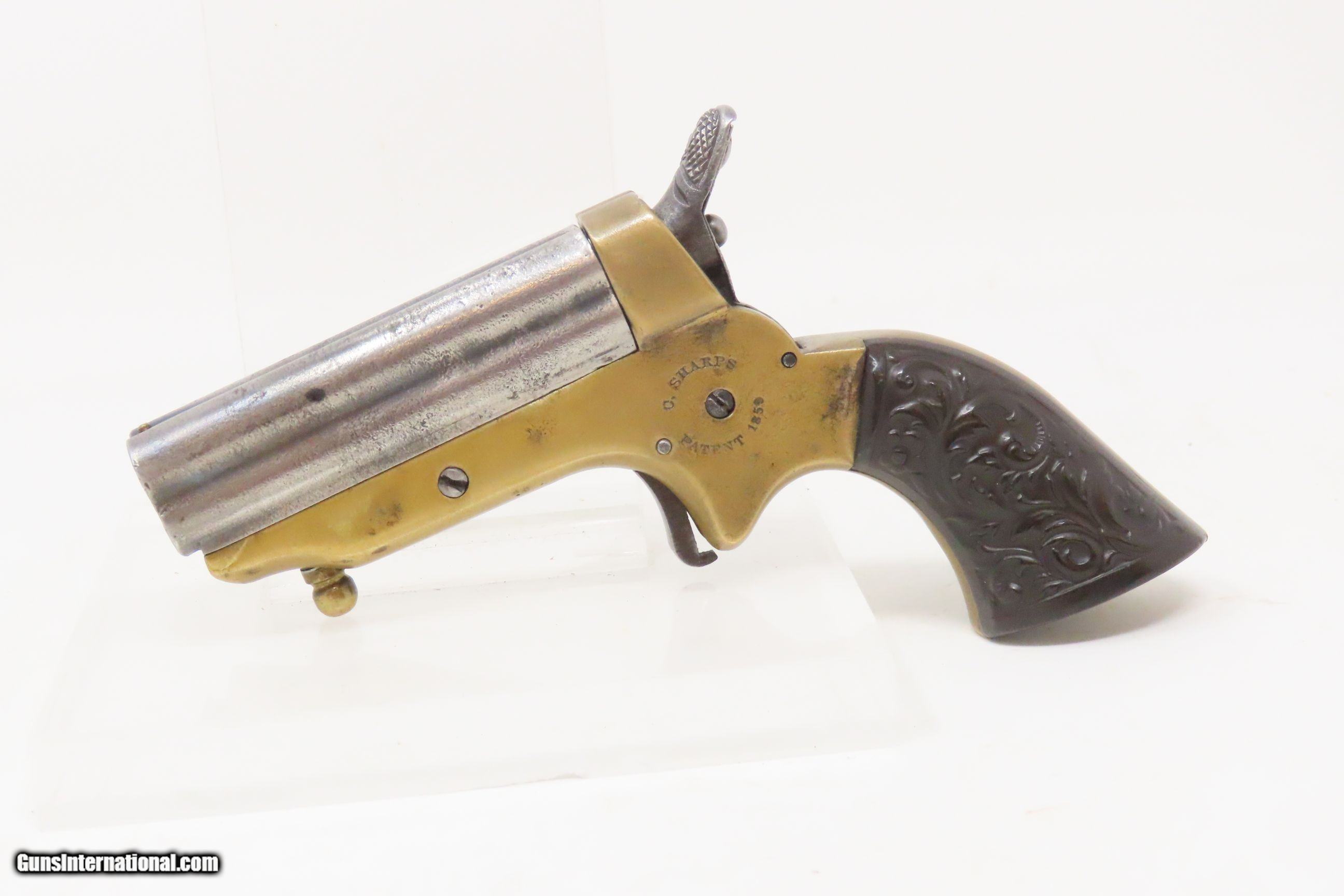The image displays an antique, well-worn pistol, showcased on a white prop that blends seamlessly with the white background. The pistol, bearing the inscription "D. Scharf's Patent 1850," features a notably short barrel, approximately two to three inches in length. The grip is crafted from a dark material, possibly hard rubber or plastic, adorned with an ornate embossed foliage pattern, suggesting intricate craftsmanship. The frame of the pistol includes small text that likely denotes the model. The barrel and hammer are made from a silver metal, and straight-head screws are visible on the frame. The gun has a single hammer and trigger in a pulled-back position, reflecting its revolver design. The overall size of the gun is around four inches, emphasizing its compact nature. Positioned within the lower-left corner of this rectangular image, the text "GunsInternational.com" appears in white with a black border. The gun's age and extensive use are evident from its aged and worn appearance.